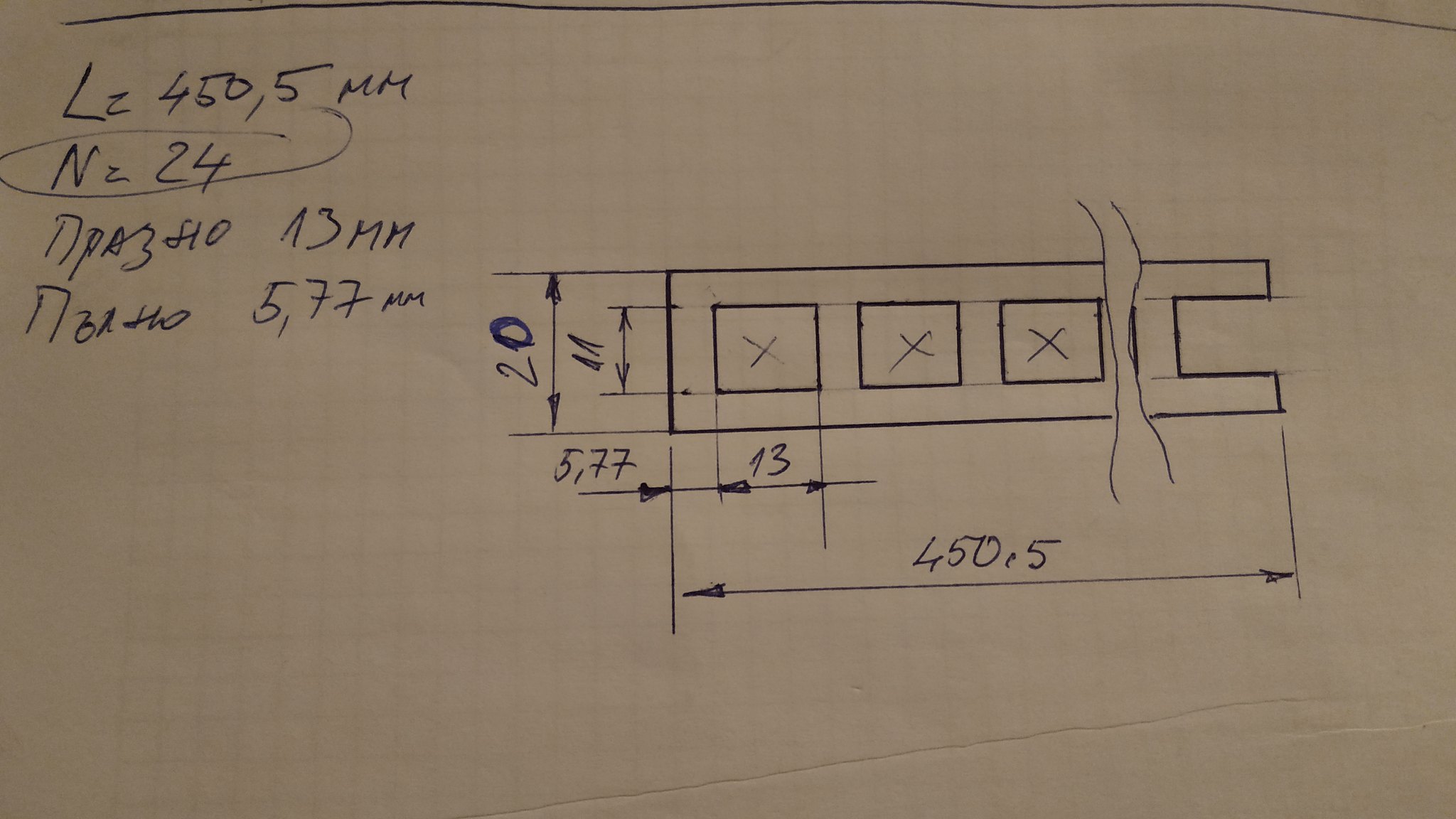The image features a detailed technical drawing on grid paper, with various labeled measurements and diagrammatic annotations. In the top left corner, the drawing lists "LZ 450,5" and "MM," surrounded by a predominantly blue ink. Central to the image is a prominent "N" located near "24," accompanied by "NCA 83HO," and the measurement "13mm" below it.

Additionally, beneath the main components, "staple 33HO" is indicated, alongside a spacing measurement of "5,77mm." On the right-hand side, there is a series of squares, each varying in size. Among these, one set of squares is labeled with "20" (with arrows pointing up and down), while a smaller set indicates "11" with similar notation. To the far right, another set of squares features X's inside, with measurements marked as "13" (arrows pointing left and right).

Adjacent to these, another measurement reads "5,77" and "22," which appears slightly misaligned. Extending horizontally across the middle of the rectangle, a label "450,5" is directed left and right, matching measurements in the top left. Notably, two wavy lines suggesting a river flow into one section on the right-hand side.

The entire drawing appears superimposed on white paper, with a background grid pattern faintly visible through the layers. At the bottom of the image, there's a noticeable scratch or indent spanning horizontally, with another element snaking in alongside it.